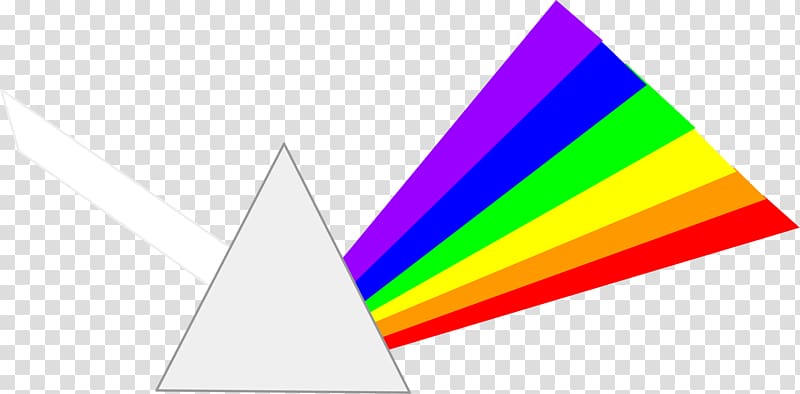This image appears to be a computer-generated graphic, possibly reminiscent of 1990s design styles. The background is marked by a white and light gray checkerboard pattern, indicating that it is a rendered image. Dominating the center-left of the frame is a light gray triangle with a black outline, its base nearly flush with the bottom of the frame. Extending from the upper left leg of the triangle is a white band angled upward at a 45-degree angle, with its far left edge almost parallel to the left edge of the frame. To the right of this triangle, a series of colored bands forms a rainbow spectrum, fanning out to the upper right. These bands, arranged from top to bottom, are purple, blue, green, yellow, orange, and red. The colors begin small and expand in size as they move outward from the triangle. This structured arrangement evokes the appearance of a prism dispersing light into its constituent colors, set against the minimalist gray and white checkered background.